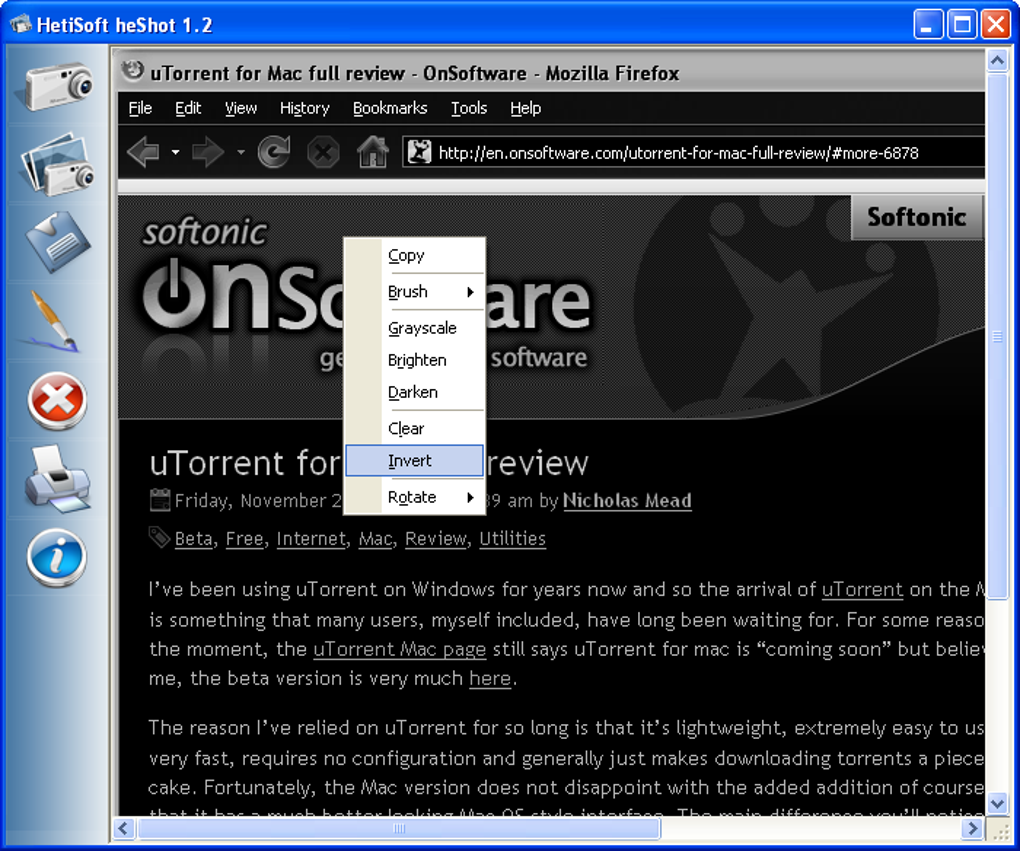Screenshot of a vintage digital environment: The image portrays a blue icon representing a digital camera alongside an outdated floppy disk – a throwback to older technology since floppy disks are no longer in use. Additionally, there are icons of a pen, stop sign, and printer. The interface has black text against a gray background, displaying "SONIC Software" and "uTorrent review." The review text mentions long-term usage of uTorrent on Windows, describing its lightweight nature and ease of use before abruptly cutting off. The pop-up menu, triggered by a right-click, lists options like copy, brush, grayscale, bright and dark adjustments, and clear. The text is styled in a distinctly retro computer font. This appears to be an old Macintosh screenshot, likely from around 1988, showcasing uTorrent for Mac in its full vintage glory.